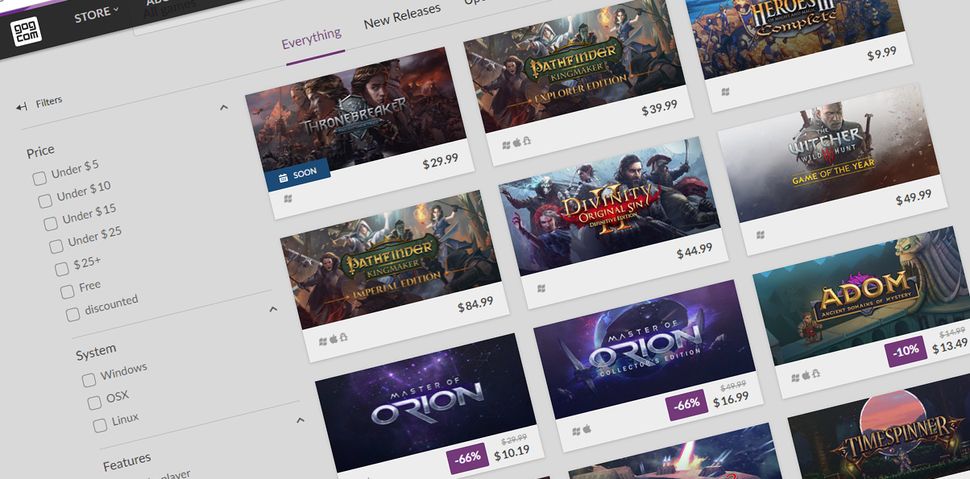At the top left corner of the webpage, "Store" appears with a drop-down menu next to "GOG.com." Down the left side, there's a series of filter options including price categories—"Under $5," "Under $10," "Under $15," "Under $25," "$25+," "Free," and "Discounted." System filters for "Windows," "OS X," and "Linux" are also present, followed by a "Features" section, although only the beginning is visible.

From left to right across the main navigation, the options visible are "Everything" and "New Releases." 

The main content includes several game listings:
1. A promotional image for "Thronebreaker" with a "Coming Soon" tag, priced at $29.99 for Windows.
2. "Pathfinder: Kingmaker, Explorer Edition," available for Windows, Apple, and Linux at $39.99.
3. "Heroes 3," exclusively for Windows.
4. "Pathfinder: Kingmaker, Imperial Edition," available for Windows, Apple, and Linux, priced at $84.99.
5. "Divinity: Original Sin 2" for Windows only, priced at $44.99.
6. An incomplete title, presumably "The Witcher: Game of the Year Edition," for Windows only.